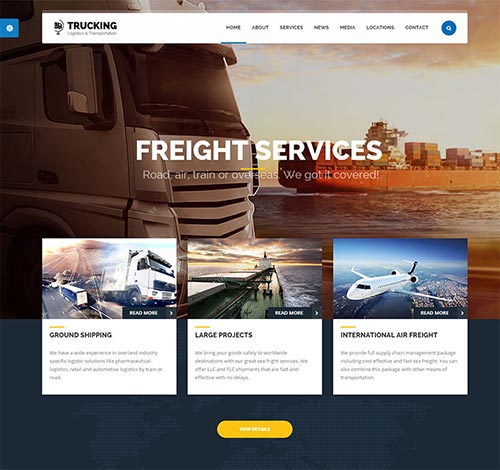**Website Homepage for a Trucking Company: Detailed Description**

The homepage of this trucking company’s website prominently features its branding and navigational elements. At the top of the page, the word "Trucking" is visible in the search bar, accompanied by a logo that depicts the front of a semi-truck with a half-circle around it. Beneath the logo, there are two additional words, too blurry to discern, all set against a dark brown color palette.

On the right side of the page, the navigation menu displays the options: Home, About, Services, News, Media, Locations, and Contact. Each of these options is written in brown with an underline highlighting the currently selected "Home" page. Adjacent to the menu is a small blue circle containing a white search icon.

The main visual on the home page features the front of a semi-truck, showing its windows and cab. In the background, there's a scene depicting water with a shipping barge, under a blue sky filled with soft white clouds. Across the middle of this image, there's a bold caption reading: "Freight Services: Road, air, train, or overseas. We've got you covered."

Below this primary image, there are three sections each featuring different transport services:

1. **Ground Shipping**
   - Image: A white semi-truck, seemingly involved in a dynamic motion.
   - Caption: "Ground Shipping" in bold black text above a short descriptive paragraph (too blurry to read).
   - Call to Action: A black banner with "Read More" in white text.

2. **Large Projects**
   - Image: A scene with water and a shipping barge in the background.
   - Caption: "Large Projects" in bold black text above a short descriptive paragraph (too blurry to read).
   - Call to Action: A black banner with "Read More" in white text.

3. **International Air Freight**
   - Image: A white airplane flying in a clear blue sky, with an aerial view of buildings and water below.
   - Caption: "International Air Freight" in bold black text above a short descriptive paragraph (too blurry to read).
   - Call to Action: A black banner with "Read More" in white text.

Finally, at the bottom of the page, there's another banner set against a black background with a gold overlay that seems to say "View something," though it is too blurry to decipher clearly.

This homepage effectively showcases the company's various freight services with corresponding images and clear call-to-action buttons, inviting users to delve deeper into each category for more information.